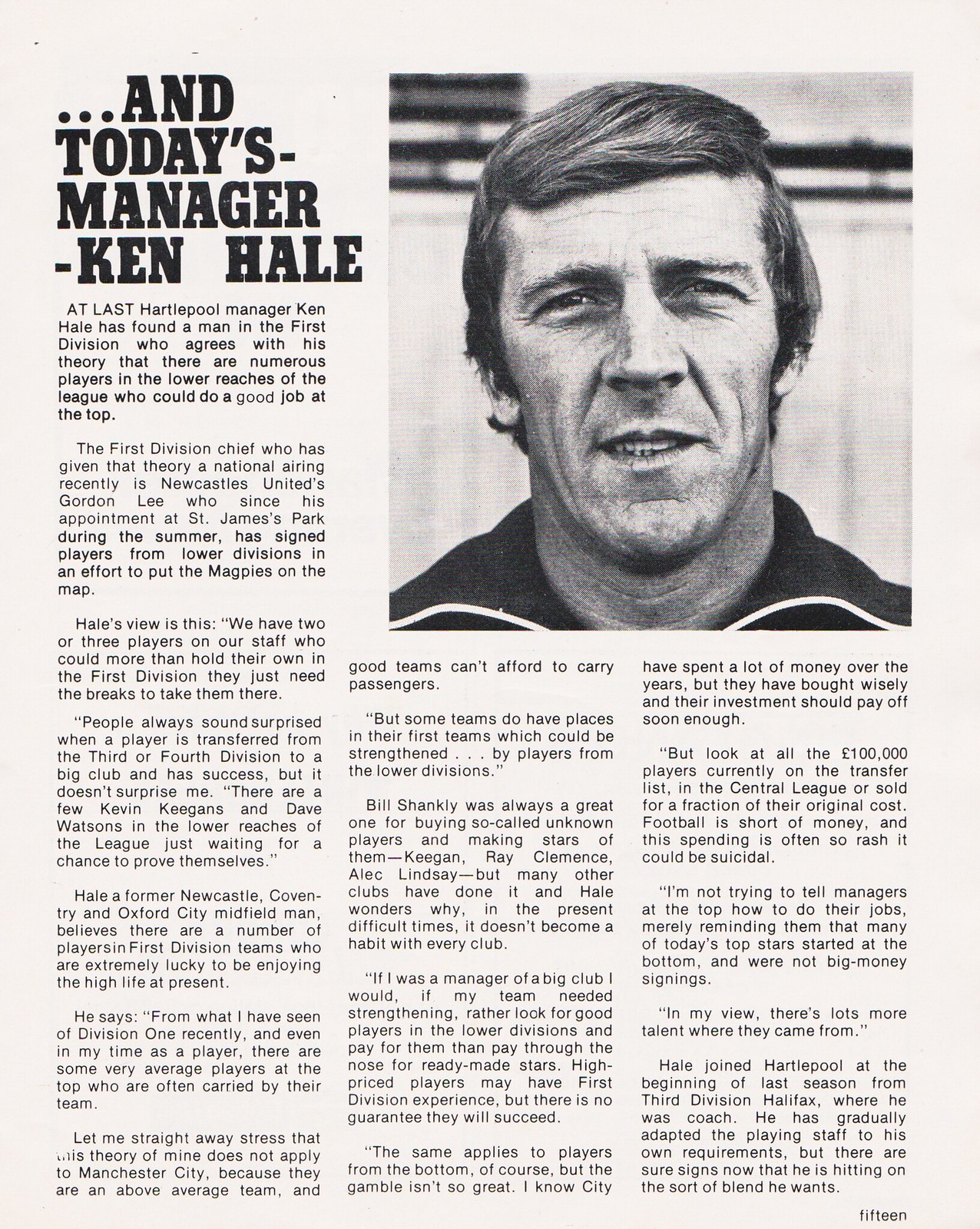This vintage magazine page, seemingly aged and on light gray paper, features an article prominently titled "...and today's manager - Ken Hale" in large bold black fonts at the top left corner. The layout includes a photograph of a clean-shaven white man with short hair, wearing a black jacket with white stripes, positioned at the top right corner. In the blurred background of the photograph, a building or wall is faintly visible. The article, arranged in three columns, discusses Hartlepool manager Ken Hale's views on scouting talent from lower divisions. Hale, a former midfielder for Newcastle, Coventry, and Oxford City, supports the idea that many capable players in the lower leagues could excel in the first division if given the chance. He points to Newcastle's Gordon Lee, who has been actively recruiting players from lower divisions since his appointment at St. James Park. Highlighting examples like Kevin Keegan and Dave Watson, Hale argues that good talent often goes unnoticed, while some current top-division players merely ride on their teams' overall strength. He stresses that Manchester City's above-average performance exempts them from his critique but advises other clubs to consider investing in promising lower-division players rather than extravagant high-priced transfers. The text underscores that Hale joined Hartlepool from third division Halifax as a coach and has been adapting the team's playing style to achieve his desired blend. The page is numbered fifteen in words at the bottom right corner, reflecting its place in the magazine.